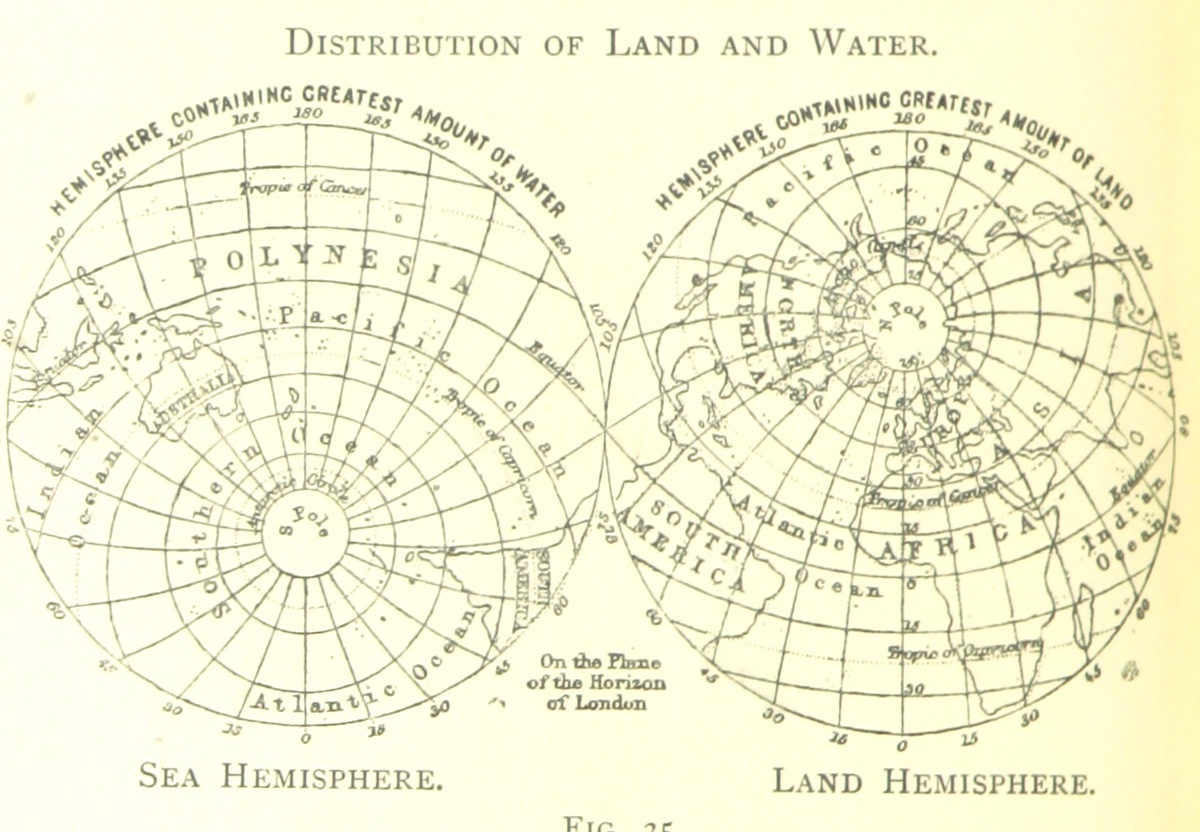The image is a vintage poster titled "Distribution of Land and Water," which prominently features two side-by-side circular drawings of the Earth. The left globe is labeled "Hemisphere Containing Greatest Amount of Water," and depicts the sea hemisphere, showcasing areas primarily dominated by oceans. Conversely, the right globe is labeled "Hemisphere Containing Greatest Amount of Land," highlighting the land hemisphere, and includes the continents of North America, South America, Africa, and Asia. Between the globes, a caption reads, "On the plane of the horizon of London." Additional annotations on the map identify various oceans and regions such as Polynesia, the Pacific Ocean, the Indian Ocean, the Atlantic Ocean, and the Southern Ocean. The poster uses a yellowish and black graphic design, rather than true photographic images. Near the bottom, it appears to have a label "Figure 25," although the number is partially cut off.